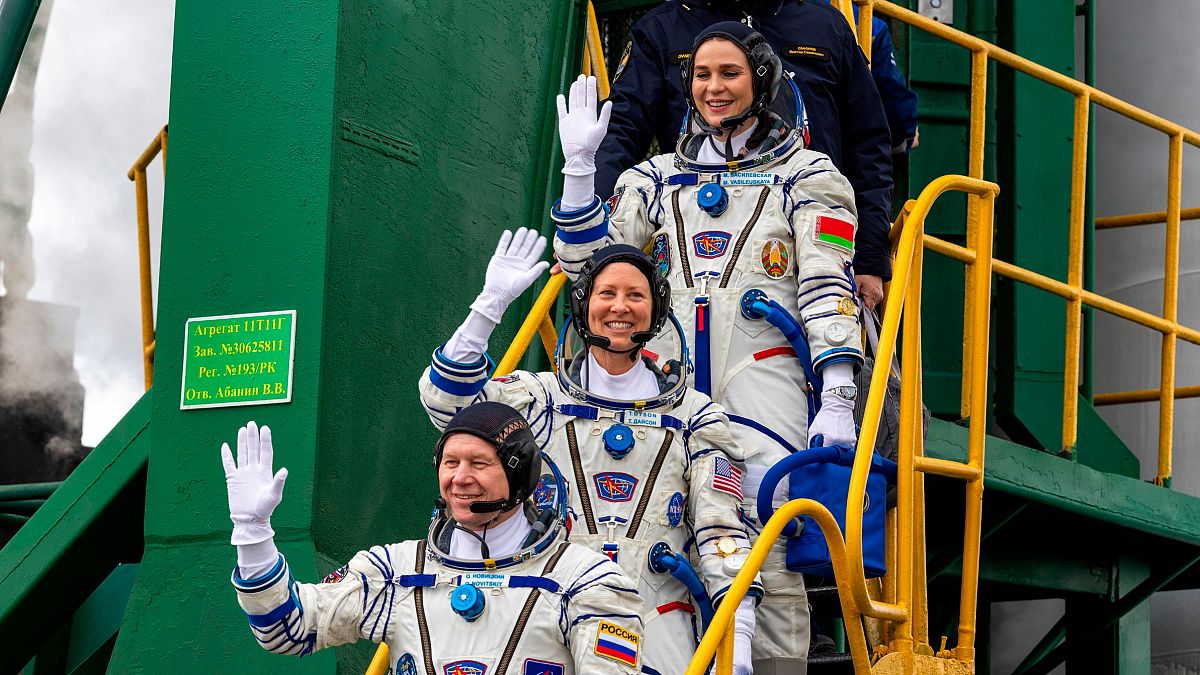The image captures a group of three astronauts descending a bright yellow metal ladder, each clad in white pressurization suits adorned with various blue-colored pipes, toggles, and instrumentation. The front astronaut, a male, is cut off from the chest upwards, visibly waving with his right hand in a white glove, and is equipped with a black helmet featuring dual microphones at the chin. The middle astronaut, a female, also waves her right hand and follows closely behind, with the third astronaut, another female, similarly waving and positioned at the top of the ladder. Each suit has a distinct country flag on the upper left arm—Polish for the front astronaut, American for the middle, and Italian for the rear. They all wear a soft-style helmet and a white turtleneck underneath their outer suit, designed with an exposed ring where a bubble-type helmet would lock on.

Behind the astronauts, partially obscured by their position, is an industrial scene featuring green crane equipment and what appears to be a sign with yellow writing, though it is not fully visible. Additionally, a figure in an official-looking dark blue jacket with yellow writing stands in the background, his face obscured from view. Together, the astronauts form a visually engaging and dynamic moment, all smiling and raised hands in unison, suggesting camaraderie and the anticipation of their mission.